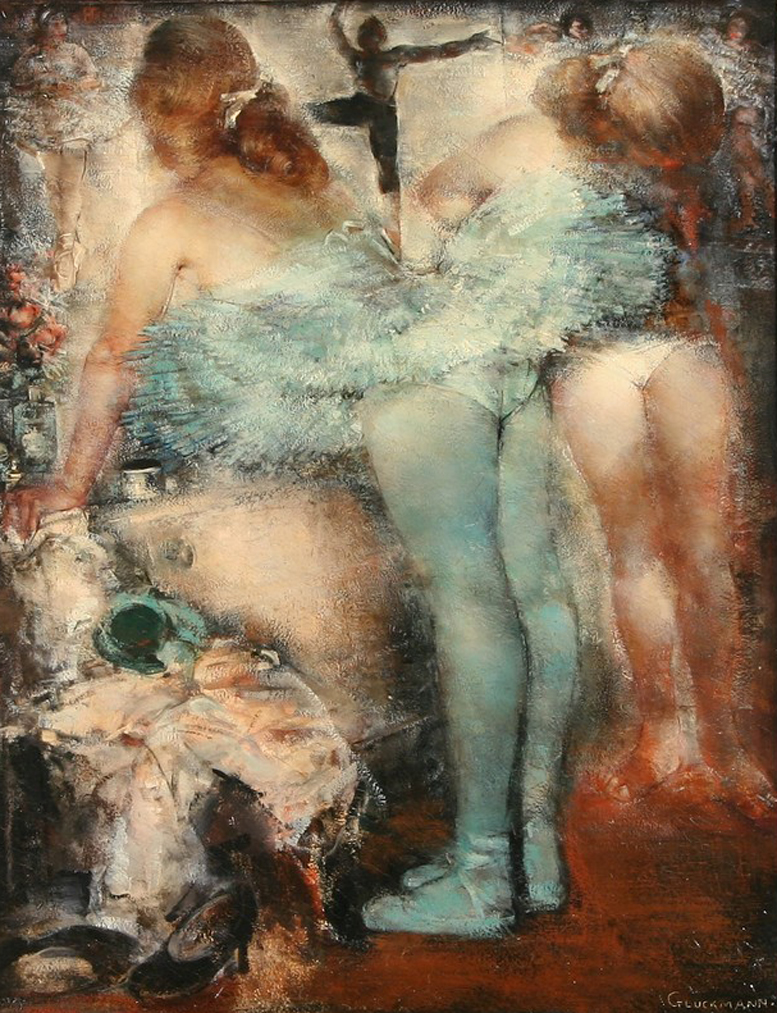The painting features predominantly red, blue, and white hues and presents multiple women, with the focal point being a ballet dancer. The central figure, a light-skinned ballerina with reddish-brown hair, is bent over with her hands on a white table, her body painted in blue, and her underwear visible. She is wearing pointe shoes and a tutu, suggesting she is either mid-performance or preparing to dance. The floor beneath her is a vibrant red, adding contrast to the scene. To her immediate left on the floor are regular shoes and clothes, indicating she has changed into her ballet attire. Surrounding this central figure are other dancers: in the top left, a woman stands; in the top middle, another woman appears to be dancing, silhouetted in black; to the right, a girl with brown hair and skin-toned legs is poised, her attire suggesting she is also preparing to dance. The background is light-colored with shades of white and gray, adding depth and a sense of space to the composition. The overall scene evokes a dynamic and preparatory atmosphere reminiscent of the works of Degas.